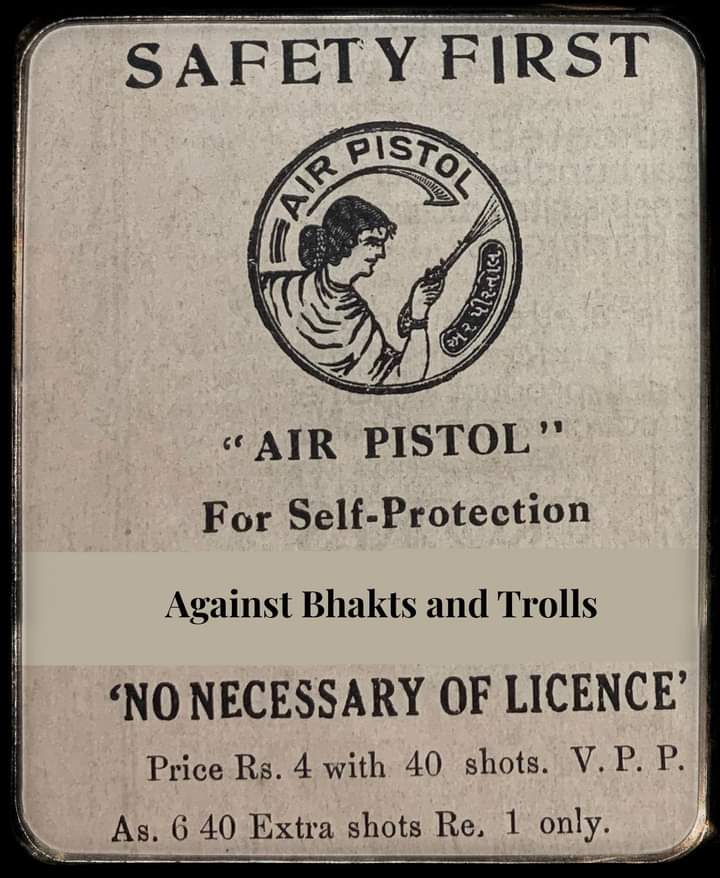This image depicts an antiquated poster or page from an old book with a white background and black lettering, promoting the use of air pistols for self-protection. The title "Safety First" is prominently displayed at the top in an interesting, uneven, and slanted font that adds to its aged appearance. Centrally featured is an emblem with a woman, her hair pulled back in a bun, pointing an air pistol. Below the emblem, it reads "air pistol for self-protection against bots and trolls," with a peculiar term "BHAKTS" mentioned. Additional text states "no necessary license," pricing as "RS4 with 40 shots," and offers "40 extra shots for 6." The overall design and wear suggest it is an old advertisement or a security poster, perhaps digitally manipulated or turned into a meme later on.